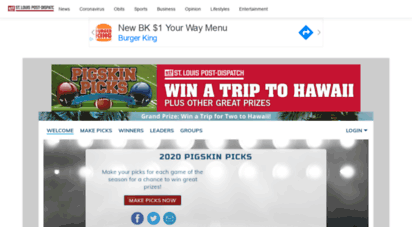The image features the iconic Burger King logo at the top, displaying a yellow bun with the "Burger King" text in red sandwiched between two yellow buns. To the right of the logo, there is a label advertising the "New BK $1 Your Way Menu" with "Burger King" written in blue text.

Below this, the text reads "Pigskin Picks," accompanied by two football helmets—one red and one blue—against a green football field backdrop complete with white yard lines. To the right, a red rectangle contains white text proclaiming "St. Louis Post Dispatch," with the bold announcement "Win a Trip to Hawaii" beneath it, followed by a smaller line reading "plus other great prizes."

The image also provides different navigation options including "Welcome," "Manage Picks," "Winners," "Leaders," and "Groups." Notably, "2020 Pigskin Picks" is inscribed in blue text. Social media sharing options are positioned at the bottom featuring icons for Facebook and Twitter, including a blue circle with a small white "F" for Facebook and a light blue circle with a white bird for Twitter.